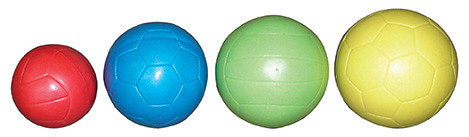This image features four balls of varying sizes and colors, arranged horizontally against a completely white, transparent, or borderless background. The balls increase in size from left to right. Starting from the left, the first ball is the smallest, a shiny red volleyball with a reflective white spot in the middle. The next ball is a slightly larger blue soccer ball, also featuring a reflective light spot. Following that is a green volleyball, which is bigger than both the red and blue balls, and lastly, the largest ball on the far right is a yellow soccer ball. All four balls exhibit a shiny surface due to light reflection, and despite some debate, they could be mistaken for candies or soap balls rather than actual sports equipment, as they sport an equally smooth and glossy finish with distinctive hexagonal patterns like those found on a soccer ball.